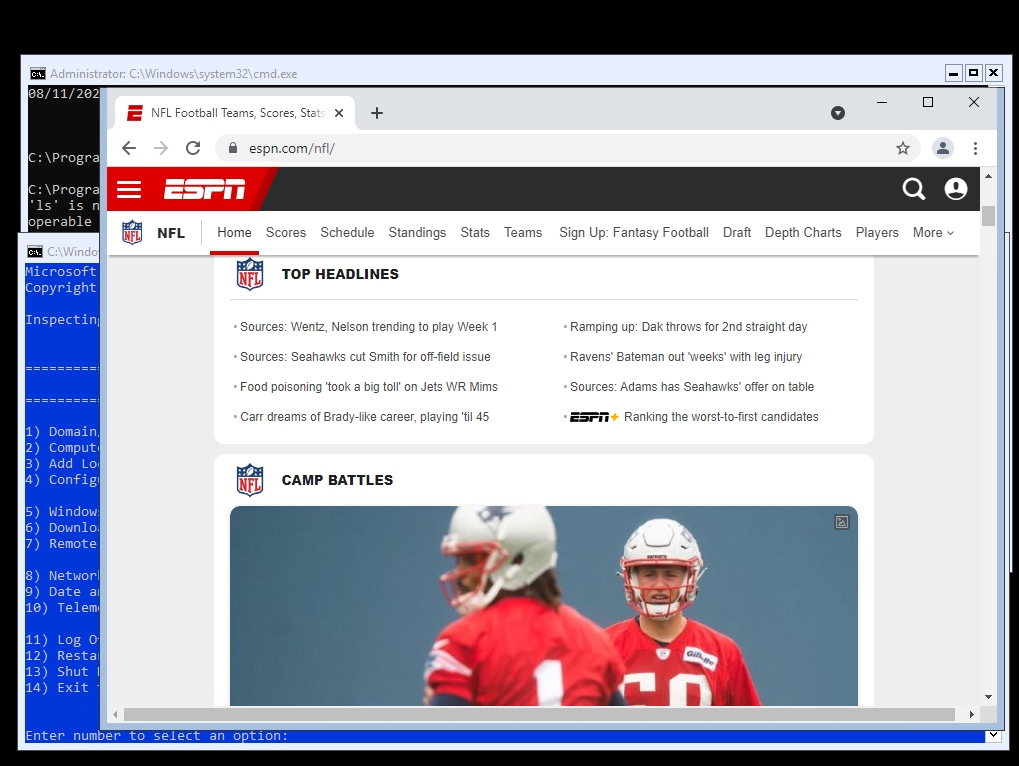In the image, there are three nested screens creating a layered effect. The topmost screen captures an ESPN webpage dedicated to NFL football. At the very top, there's a tab displaying the ESPN logo, a cancel icon, and several other elements such as a search bar with the URL "ESPN.com/NFL", a profile icon, a favorites icon, a reload icon, and a more icon. Below this is a horizontal black bar with a search icon and another generic profile icon.

Moving down the page, the ESPN logo appears prominently in red, beneath which is a horizontal menu featuring multiple options—NFL logo, Home, Scores, Schedule, Standings, Stats, Teams, Sign-up, Fantasy, Draft, Depth Charts, Players, and a More tab. 

Further down, the section titled "NFL Top Headlines" appears with bullet points for various stories. The headlines include: "Sources: Wentz, Nelson trending to play Week 1", "Food poisoning took a big toll on Jets WR Mims", and "Carr dreams of Brady-led career, playing until 45." Lastly, an article about "Camp Battles" is shown, accompanied by an image with the NFL logo to the left.

The layers of the screen capture emphasize the different functional elements of the ESPN webpage, while the detailed headlines and structured sections provide a comprehensive snapshot of the NFL-focused content.